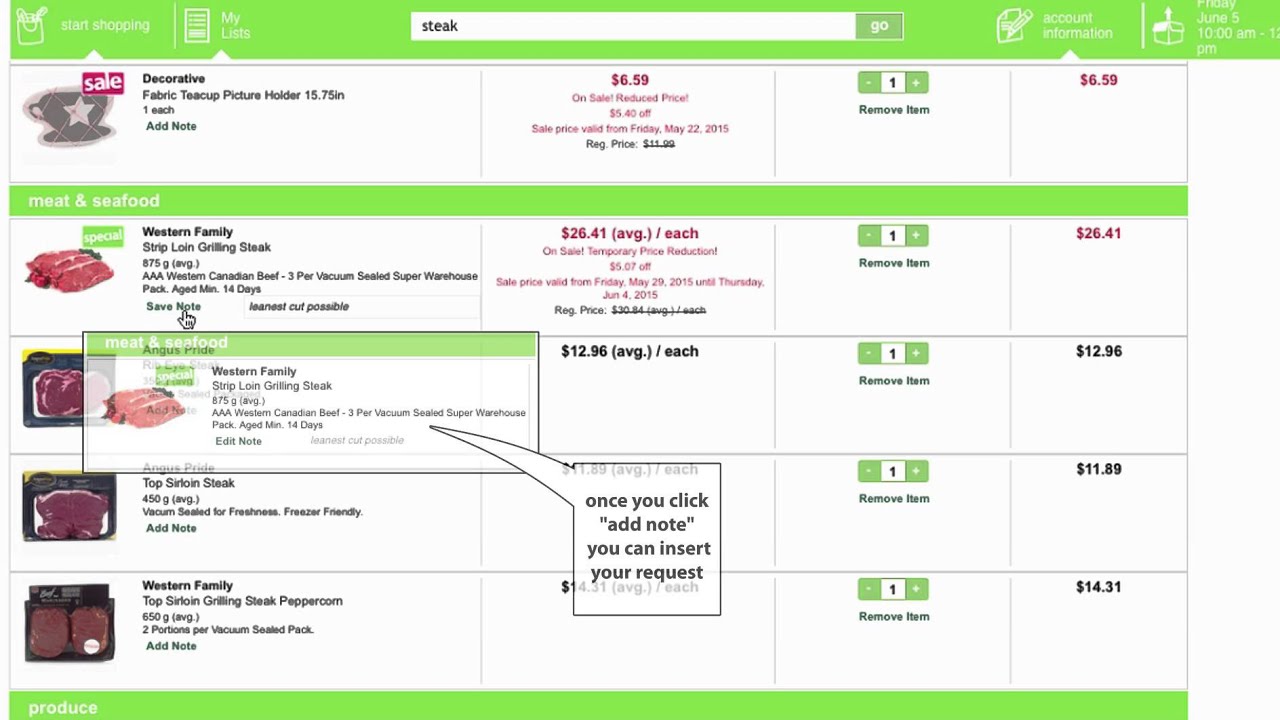This image is a screenshot of a grocery store's online shopping interface, specifically showcasing the meat and seafood section. The background is predominantly white, with a lime green navigation bar at the top. On the left side, there's a small clipart image of a shopping bag next to the text "Start Shopping." Below this, another clipart image displays a list with the text "My Lists." 

In the central area, there's a white search box containing the word "steak" in black lettering, accompanied by a green rectangular button with the word "Go" in white text. To the right, account information is displayed, including a scheduled delivery time: "Friday, June 5th, 10 a.m. to 1 p.m."

Directly below, a red "Sale" label with white letters catches the eye. Adjacent to this is a description reading "Decorative fabric teacup picture hidden, 15.75 M, one each," priced at $6.59, highlighted in red to indicate the sale price. To the right of this description is a quantity adjustment feature, with a green minus and plus sign allowing the user to modify the quantity. The adjusted price is displayed again to its right.

The section beneath showcases four different types of steaks available for purchase. Each steak listing includes the cost, a section for quantity adjustment (featuring remove, increase, or decrease options in green), and the respective price.

At the bottom of the screen, a green bar labeled "Produce" marks the transition to another section of the grocery store.